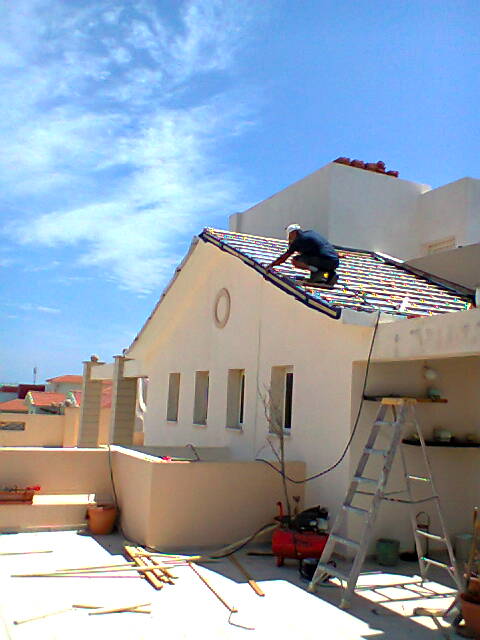This intriguing image captures a man diligently working on the roof of a beige, Mesa-style house with smooth walls and marked by a sunlit, arid landscape. The house features four clearly cut windows on the left side, which face a flat area that could be a parking lot or storage space. Prominently situated in the right foreground, a roughly four-foot-tall fence extends from the back of the house, leading towards an open area that contains various objects including a red machine and a wheelbarrow positioned in the bottom right corner.

The man on the roof, who is wearing a dark blue shirt, blue shorts, white socks and tennis shoes, and a white hat, is captured working with what appears to be a power tool connected via a cord that extends to his location. His back is turned to the camera, obscuring his identity and age. The roof itself is peculiar, adorned with multicolored specks resembling leaves or Christmas lights in blue, red, and gray hues.

An older ladder with paint drippings and signs of extensive use, which the man presumably used to ascend to the roof, leans against the house near a garage bay. The sunny weather and clear blue sky peppered with white clouds cast a bright ambiance over the scene, and in the distance, a few neighboring houses and their roofs are visible, enhancing the sense of locale and environment.